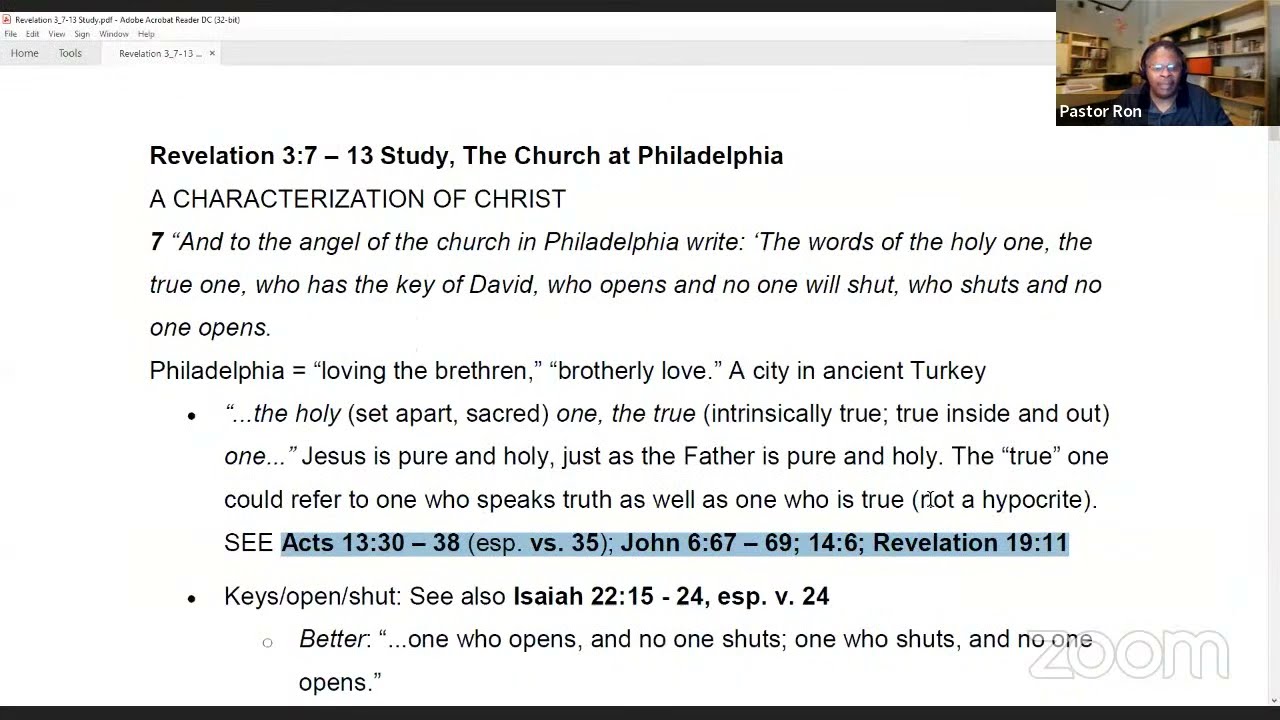The image is a screenshot of a Zoom call featuring a religious study group led by Pastor Ron, a bespectacled African American man donning a headset, a collared shirt, and possibly a dark cardigan. In the top right corner, a small box displays Pastor Ron sitting at a computer desk with shelves and various items in the background. His name is clearly visible at the lower corner of his image. The main screen shows a white page with black text that reads: "Revelation 3:7-13 Study, The Church of Philadelphia." Below that, the title "A Characterization of Christ" is visible. The text continues with a passage explaining Christ's attributes and references to other Biblical verses, such as Acts 13:30-38 and John 6:6-9. Prominently highlighted is a description of Philadelphia, known for brotherly love, and an interpretation of Christ as "The Holy One" and "The True One." This intricate background and detailed scripture emphasize the session's focus on the deep study of the Bible, particularly regarding Christ's depiction and teachings in the context of the Church at Philadelphia.